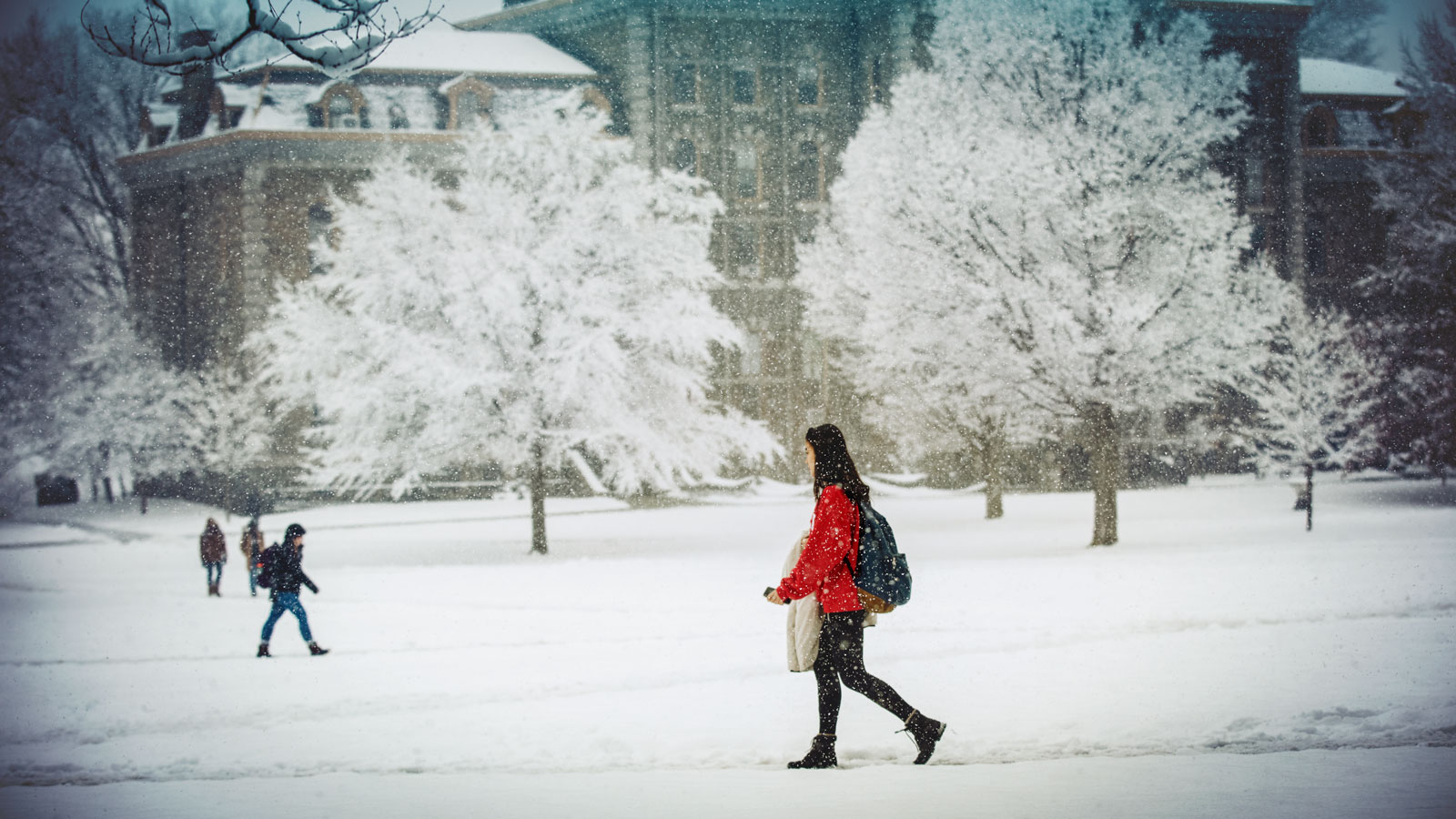In this detailed illustration of a snowy winter scene on what is likely a college campus, four students are making their way through snow-covered pathways and fields. In the foreground, a young woman with long brown hair is walking, dressed in black pants and boots, a bright red coat, and carrying a white jacket in her hands along with a dark backpack. To her left, another person is visible, cloaked in a black snow coat with a hood over their head, also carrying a backpack. In the background, two more individuals can be seen traversing the snowy landscape, likely students as well, given the context and their backpacks. The ground and trees are blanketed in approximately three inches of snow, and large snowflakes are visibly falling. Adding an atmospheric touch, a grand antique building with a brown, old architectural design stands behind the courtyard, its roof similarly covered in snow.